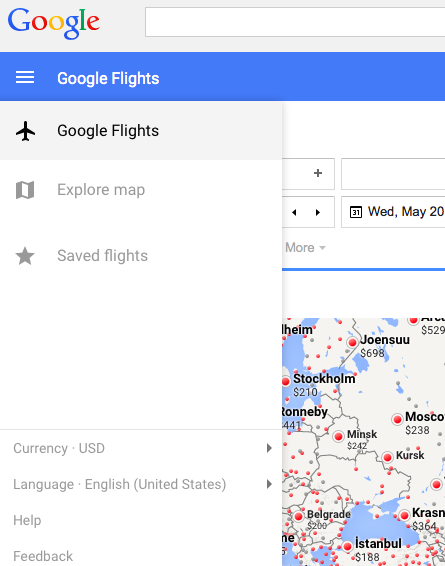The image displays a screenshot of the sidebar from Google Flights. At the very top left, the recognizable Google logo is visible. Below the logo, the menu lists various options: "Google Flights," repeated twice for emphasis, followed by "Explore Map," "Saved Flights," "Currency: USD," and "Language: English (United States)." At the bottom of the sidebar, there are links for "Help" and "Feedback." On the right side of the image, part of the interactive map feature is visible, showing locations including Stockholm, Moscow, and Istanbul.